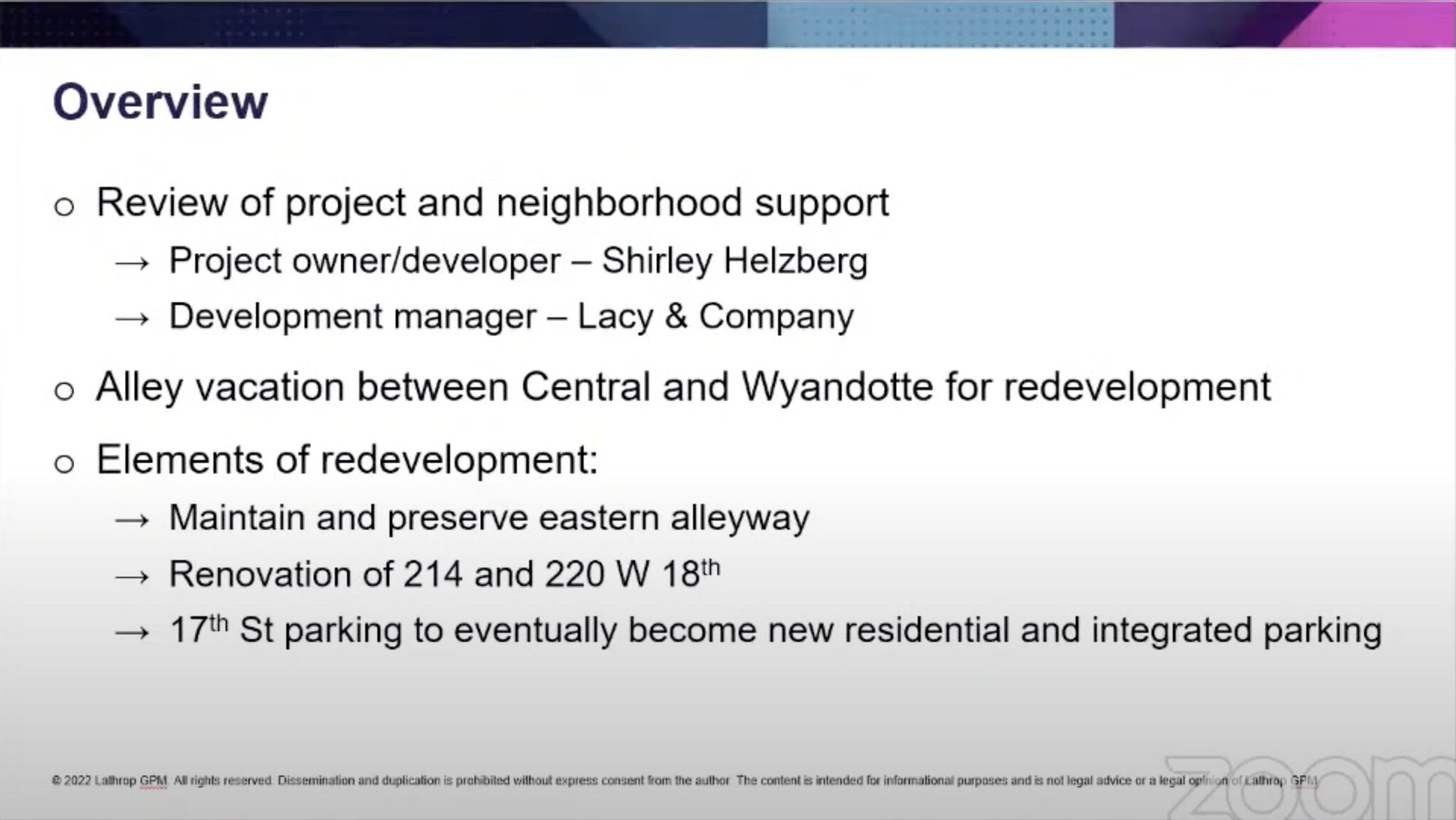This image is a detailed screenshot from a Zoom meeting, featuring a landscape-oriented PowerPoint slide. The slide has a decorative top border that transitions from black to shades of blue, light blue, purple, and pink. The main background is light gray. Positioned in the upper left corner, the word "Overview" appears in bold black print. Below it are three main bullet points:

1. **Review of Project and Neighborhood Support**:
   - Project Owner/Developer: Shirley Helzberg
   - Development Manager: Lacey and Company

2. **Alley Vacation between Central and Wyandotte for Redevelopment**

3. **Elements of Redevelopment**:
   - Maintain and Preserve Eastern Alleyway
   - Renovation of 214 and 220 West 18th
   - 17th Street Parking to Eventually Become New Residential and Integrated Parking

At the bottom, there is a copyright notice: "2022 Lanthrope GPM. All Rights Reserved. Dissemination and Duplication is Prohibited without Express Consent from the Author. The Content is Intended for Informational Purposes and is Not Legal Advice or Legal Option". This text is slightly obscured by a transparent gray Zoom watermark on the bottom right corner. The dominant colors of the slide are black, white, and gray with accents of purple and blue in the top border.